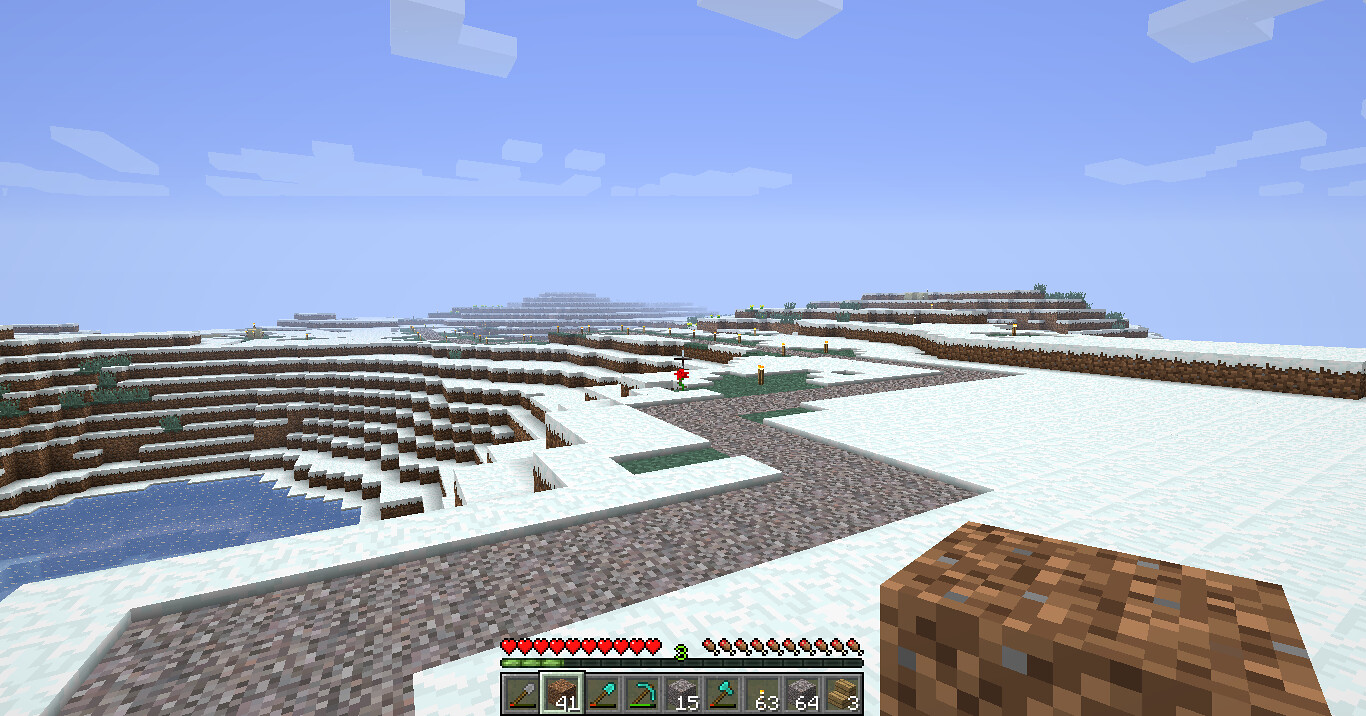This detailed screenshot from Minecraft showcases a first-person perspective view under a predominantly blue sky scattered with a few blocky white clouds. The scene features a medium to dark blue pond to the left, adjacent to a staggered hillside consisting of brown dirt patches topped with white snow and occasional green grass patches. Further accentuating the wintry environment, a gravel or stone pathway meanders through the snow, brightly illuminated by torches. The interface displays the player's health icons represented by hearts, food icons reflecting hunger levels, tools in the toolbar including a stone, wood, axe, pickaxe, and shovel, as well as an inventory count showing 45 bricks and 63 gold.